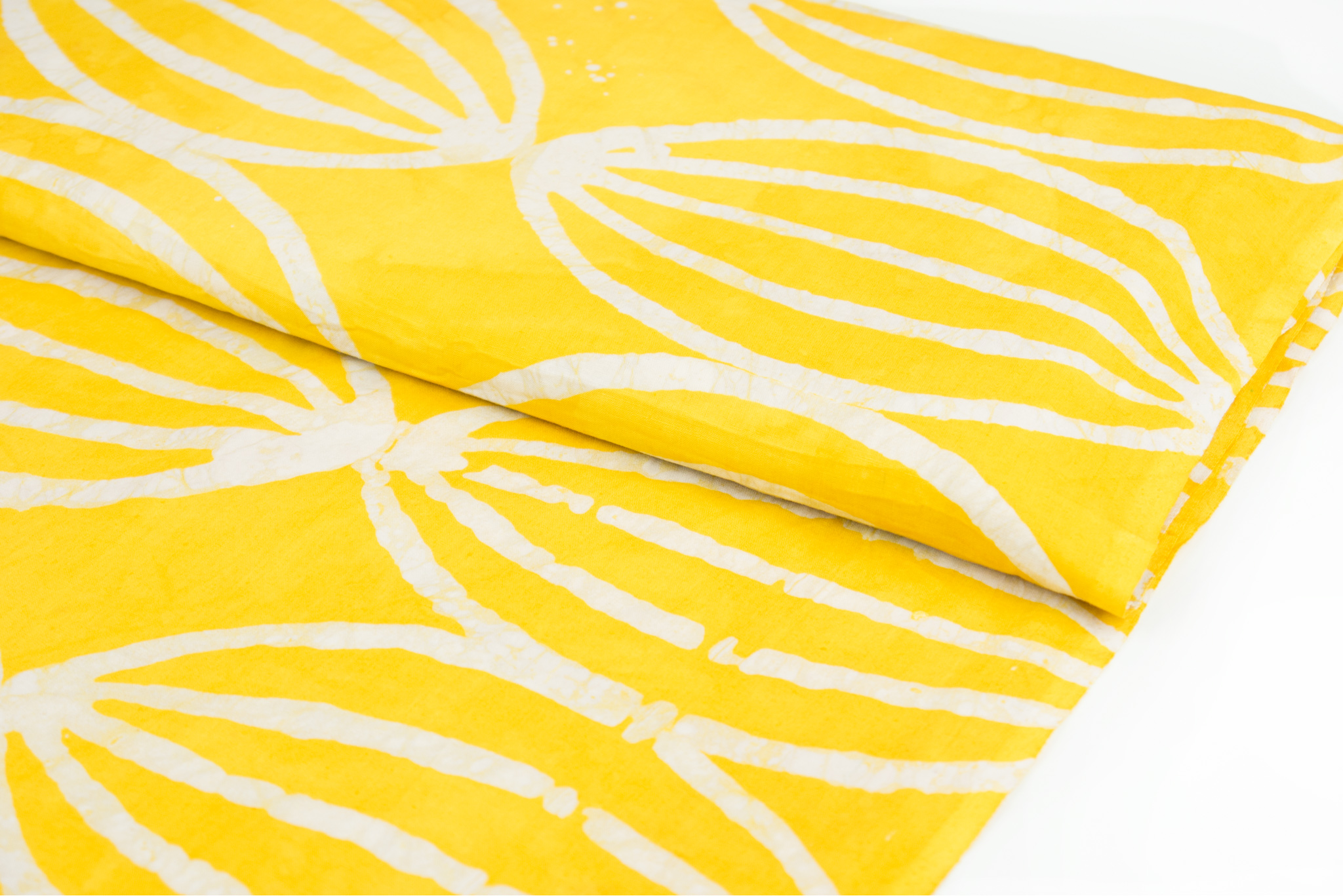The image depicts a neatly folded tablecloth made from high-quality, bright yellow fabric. The tablecloth features a sophisticated design of repeating almond-shaped patterns, each formed by five white lines, with three additional lines connecting at the central points of the shapes. The fabric, elegantly folded in a three-fold style, rests on a featureless, solid white surface—likely a countertop or table—showcasing its intricate design and vibrant color. There are no visible markings or inscriptions on the fabric.